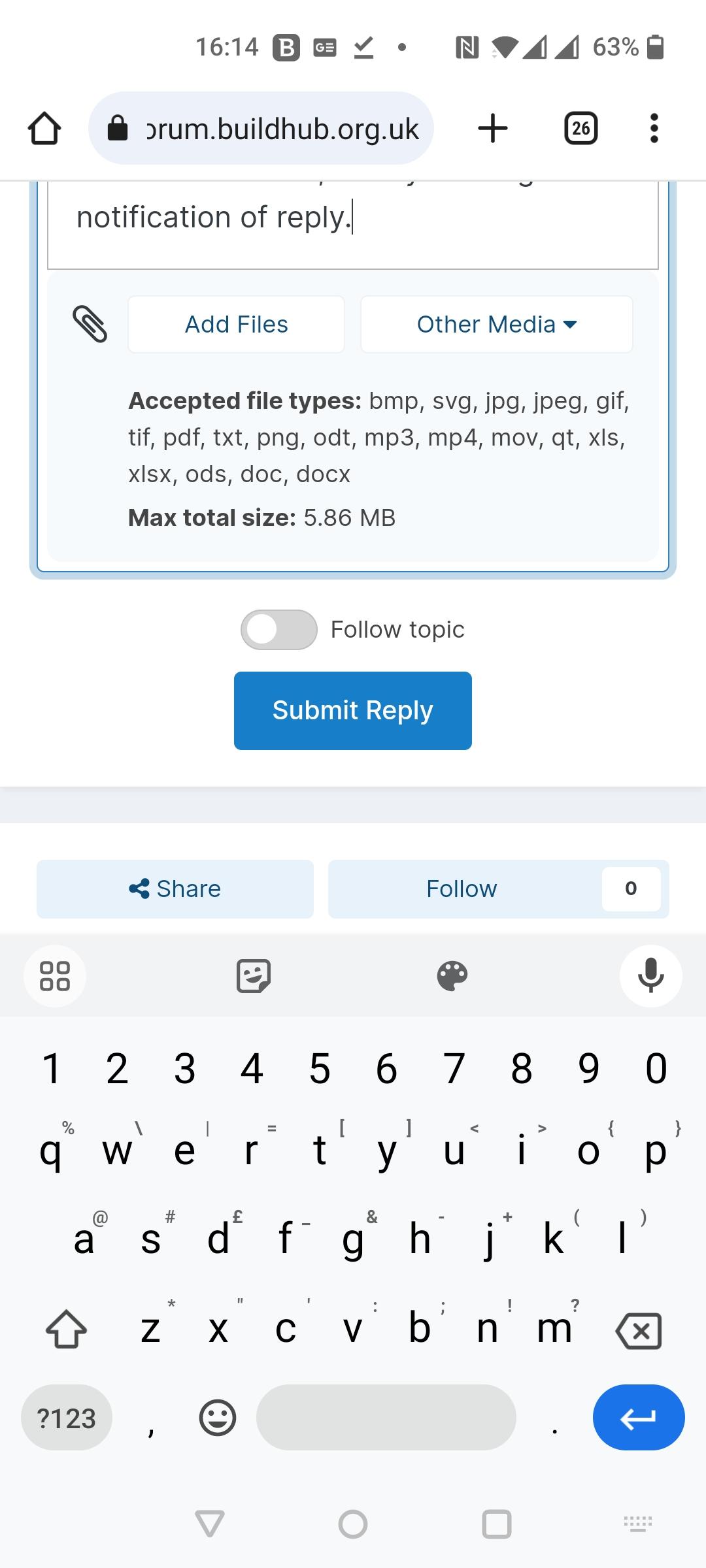A detailed caption for the image could be:

"An image of a mobile phone screen showcasing an active forum on forumbuildhub.org.uk. At the top of the screen, the device's status bar displays the time, battery level, and signal strength. The search bar is partially visible, with the text 'forum' clearly seen, suggesting it is associated with forumbuildhub.org.uk. Below the search bar, there is a forum window displaying a notification of a reply about acceptable file types. It indicates that HEAD files and other media, excluding bitmap and JPEG formats, can be uploaded, with a maximum file size of 5.86 megabytes. The lower part of the screen features an on-screen keyboard, signaling an ongoing reply. Additionally, the interface notes 26 messages in the thread and includes options to add various types of media. No fingers are visible in the picture, emphasizing the focus on the interface and the user's interaction with the forum."